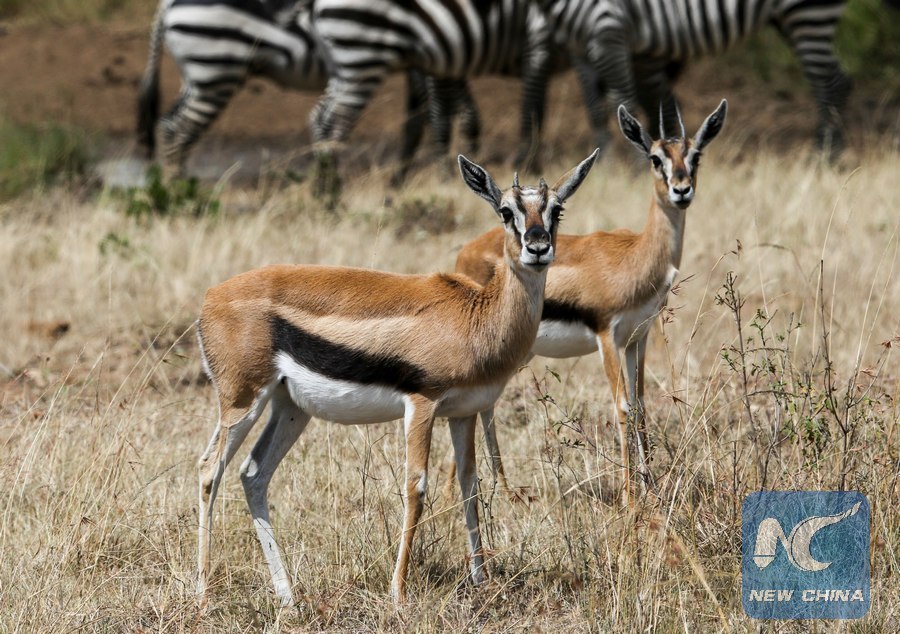In this brightly sunlit outdoor photograph, two gazelles stand amidst tall, predominantly brown brush interspersed with hints of green. The foreground, which is in sharp focus, captures the detailed texture of the gazelles' fur – a rich brown paired with distinctive black stripes and contrasting white bellies. Their slender legs and long ears give them an elegant appearance, with one standing slightly behind the other. In the softer, blurred background, three zebras stand side by side, their black-and-white striped bodies partially visible. The gazelles, which sport small horns, gaze directly at the viewer, their presence beautifully highlighted by the sunlight. A translucent "New China" logo, with artistically crafted 'N' and 'C' letters, subtly adorns the bottom right corner of the image.